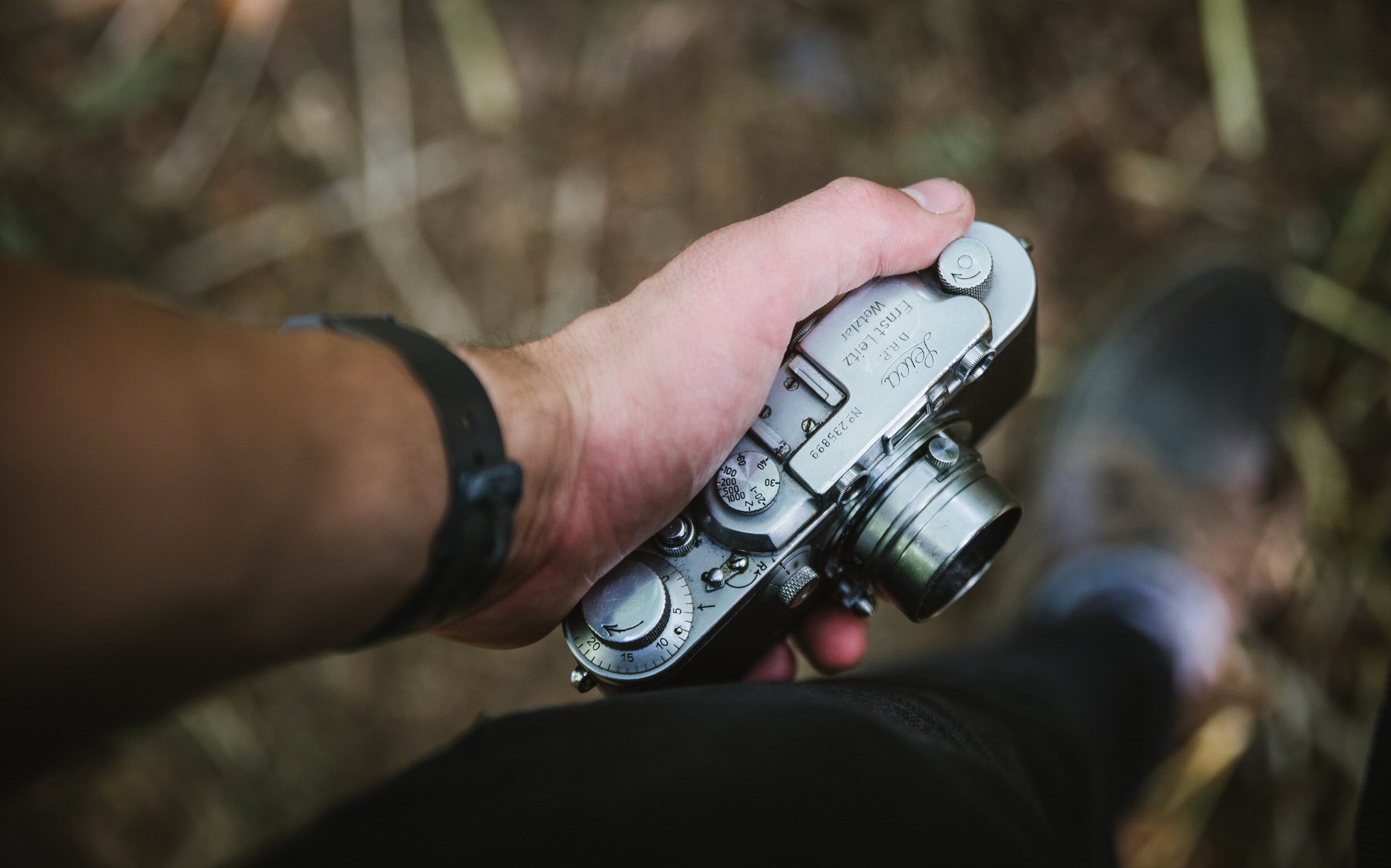The photograph, taken from an overhead perspective, captures the forearm and hand of a man gripping a vintage silver metallic camera, identifiable as a Leica due to the inscriptions "Leica" and "Ernst Weitz Wetzler No. 235899" visible on it. The camera features several dials and knobs for various settings. The man's hand, fair-skinned and adorned with a black wristwatch, is the central point of focus in the image. The background is blurred, revealing indistinct patches of dirt, green foliage, and a faint outline of the man's left foot in a black shoe wearing black pants. The entire scene exudes a timeless quality, emphasizing the detailed craftsmanship of the camera amidst the softly blurred natural surroundings.